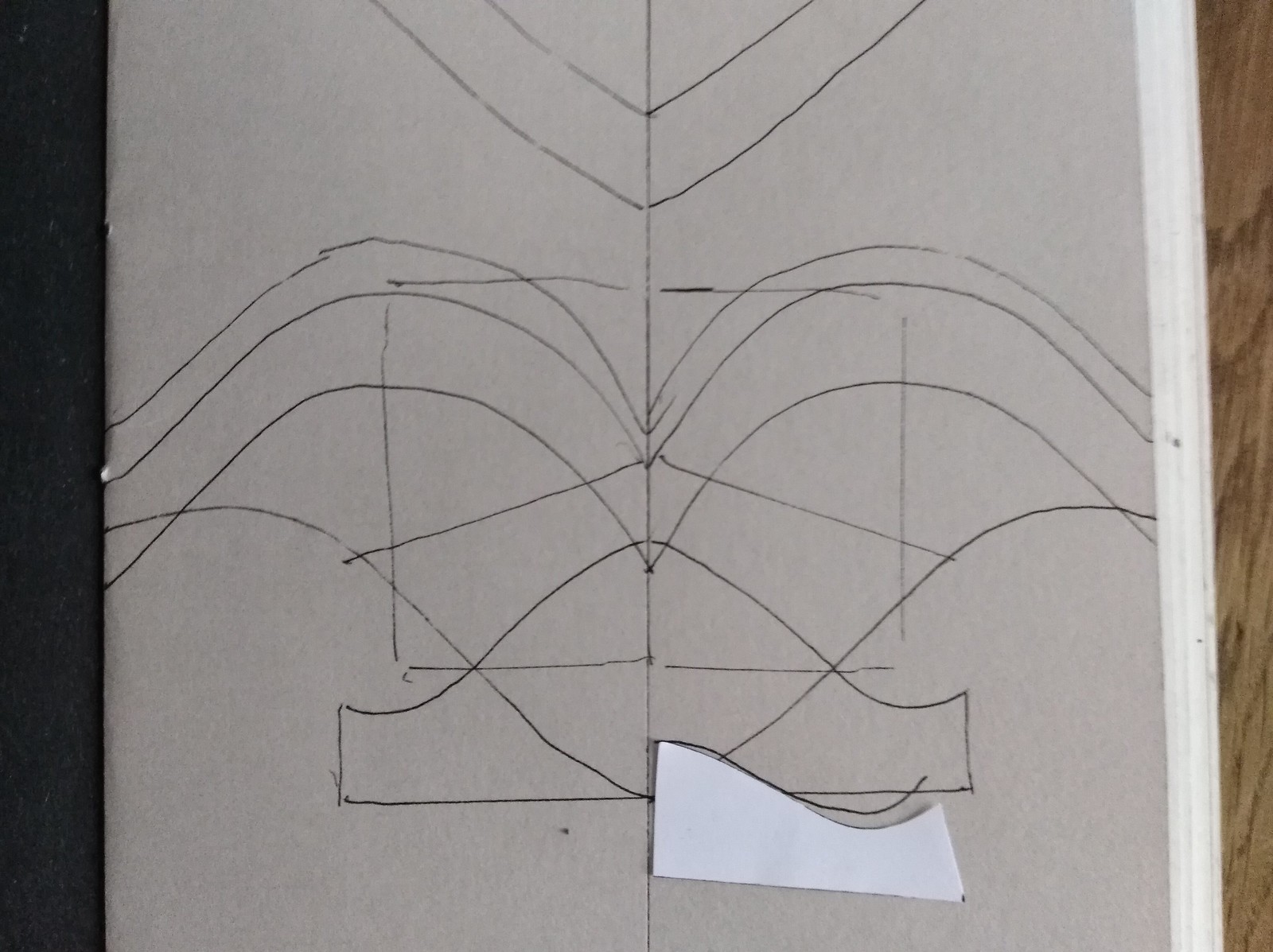The image features a piece of white paper with intricate black ink drawings. A straight line runs down the center of the paper, creating a symmetrical design where each side mirrors the other. On both sides of the central line, there are two parallel lines and various geometric shapes, including a square in the middle. The intricate patterns include additional lines and shapes that precisely reflect each other, maintaining near-perfect symmetry. In the lower right corner of the paper, there is a small, distinct piece of paper whose shape and placement align harmoniously with the overall design. The detailed drawings and balanced layout create a visually captivating and meticulously structured composition.